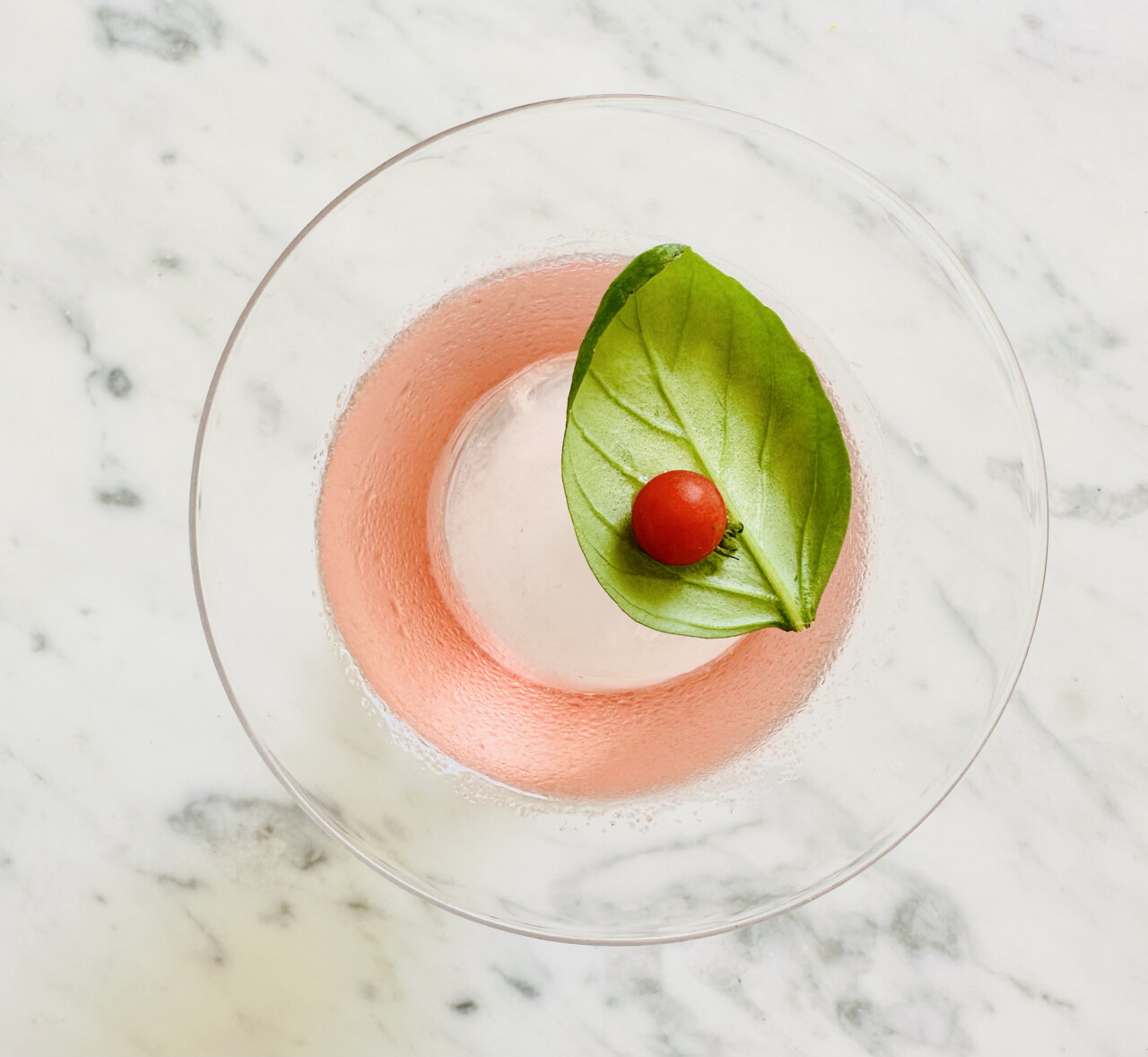The image is a high-class, food-type photograph taken from above, featuring a clear glass plate with a delicate pink rim placed on a white granite countertop with light gray swirls. At the center of the plate, a large green leaf, likely spinach, serves as a bed for a small cherry tomato. The tomato, with its green top pointing downwards, adds a pop of color to the minimalist presentation. The glass plate is slightly covered in condensation, making it appear "sweaty" and giving it a fresh, appealing look reminiscent of a high-end restaurant setting. The overall composition is simple yet aesthetically intriguing, highlighting the contrast and harmony between the elements.